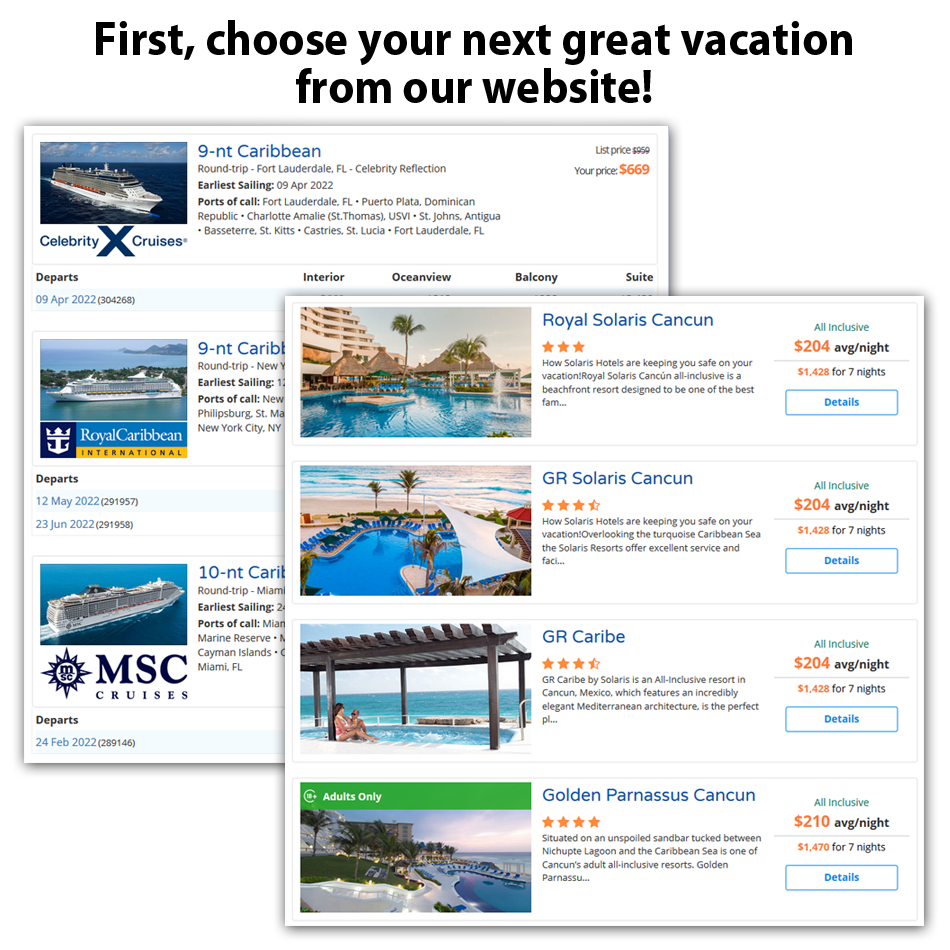This image appears to be an advertisement, likely from a website, presented on a white background. At the top, the text in large, bold black letters reads, "First, choose your next great vacation from our website."

The advertisement is divided into two main rectangular sections, slightly overlapping, with the second section positioned lower and to the right of the first. The lower section contains information about cruise deals, highlighted by three rows, though two rows are partially obscured by the section above. The bottom row is fully visible, displaying the following offer: "9NT Caribbean, priced at $669," featuring cruises from Royal Caribbean and MSC Cruises.

The upper section focuses on hotel accommodations, arranged in four rows. Each row showcases a different hotel in Cancun, along with a visual and price per night:

1. Royal Solaris Cancun: $204 average per night, with an accompanying image.
2. GR Solaris Cancun: $204 average per night, featuring a picture of a swimming pool.
3. GR Carib: $204 average per night, showing people sitting near a pool by the ocean under a pergola.
4. Golden Parnassus Cancun: $210 average per night, with a picture of a cityscape near the ocean.

This detailed layout provides a variety of options for potential travelers, emphasizing both cruising and hotel stays in exotic destinations.